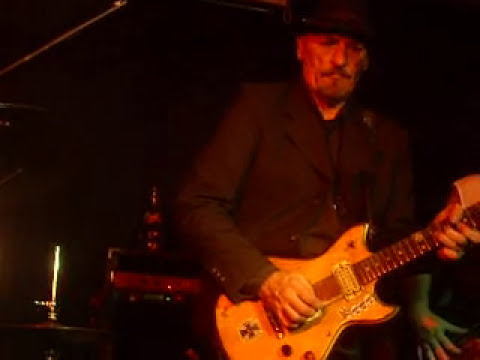In this atmospheric photo, likely taken inside a nightclub, bar, or concert hall, an older white gentleman is captured mid-performance. He exudes a serious and intense aura with his stern expression, accentuated by a mustache and goatee. His attire is dark, comprising a black suit jacket over a similarly dark shirt, and topped off with a black hat. The man is showcased under focused lighting, which illuminates him and the electric guitar he's playing—an instrument that stands out with its brown or orange hue and distinctive cross decal near the bottom.

Despite the overall darkness and low quality of the photo, details such as a speaker with a beer bottle atop it can be discerned in the backdrop, hinting at a live stage performance. Another person, barely visible, is present in the background with their hand illuminated by blue light, which adds to the scene's dynamic feel. A small beam of yellow light also punctuates the otherwise black background, subtly enhancing the image's depth and ambiance.